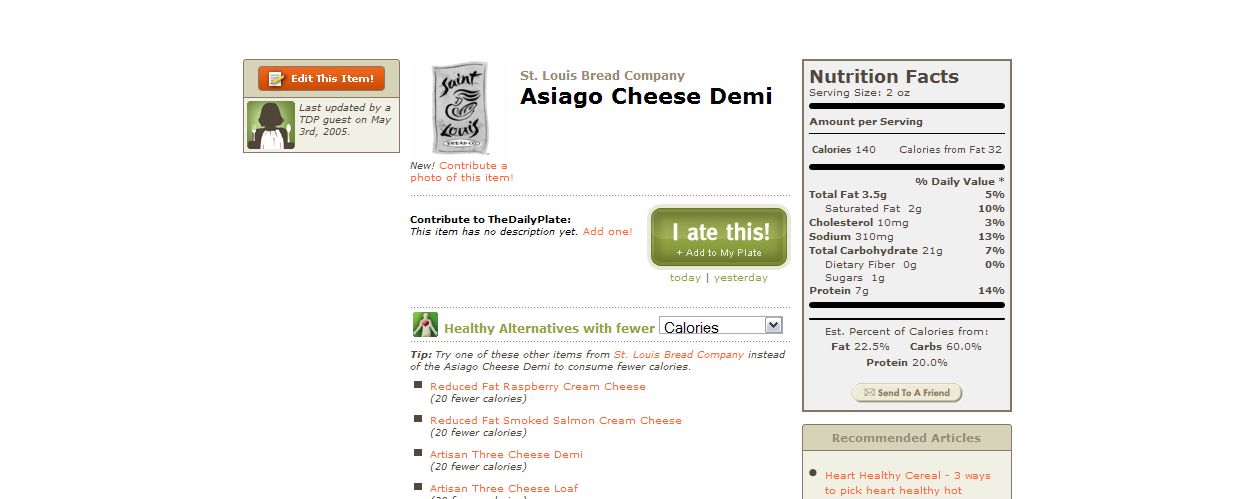The image is a detailed screenshot from a website, likely a forum or food tracking platform, displayed on a white background. In the center of the frame, the heading "St. Louis Bread Company, Asiago Cheese Demi" is prominently featured. Beneath this, a green button labeled "I ate this" invites users to add this item to their daily plate. The left panel features an orange "Edit this item" button and indicates that the page was last updated by a TDP guest on May 3rd, 2005. The right panel presents a detailed nutritional facts box, which outlines the serving size (two ounces) and the amounts of calories, total fat, cholesterol, sodium, total carbohydrates, and protein. The bottom section offers "Healthy alternatives with fewer calories" and provides a dropdown menu for easier selection. Additional links and suggestions for alternative items with fewer calories are also visible. In the bottom right corner, recommended articles with titles such as "Heart Healthy Cereal" are available for further reading.